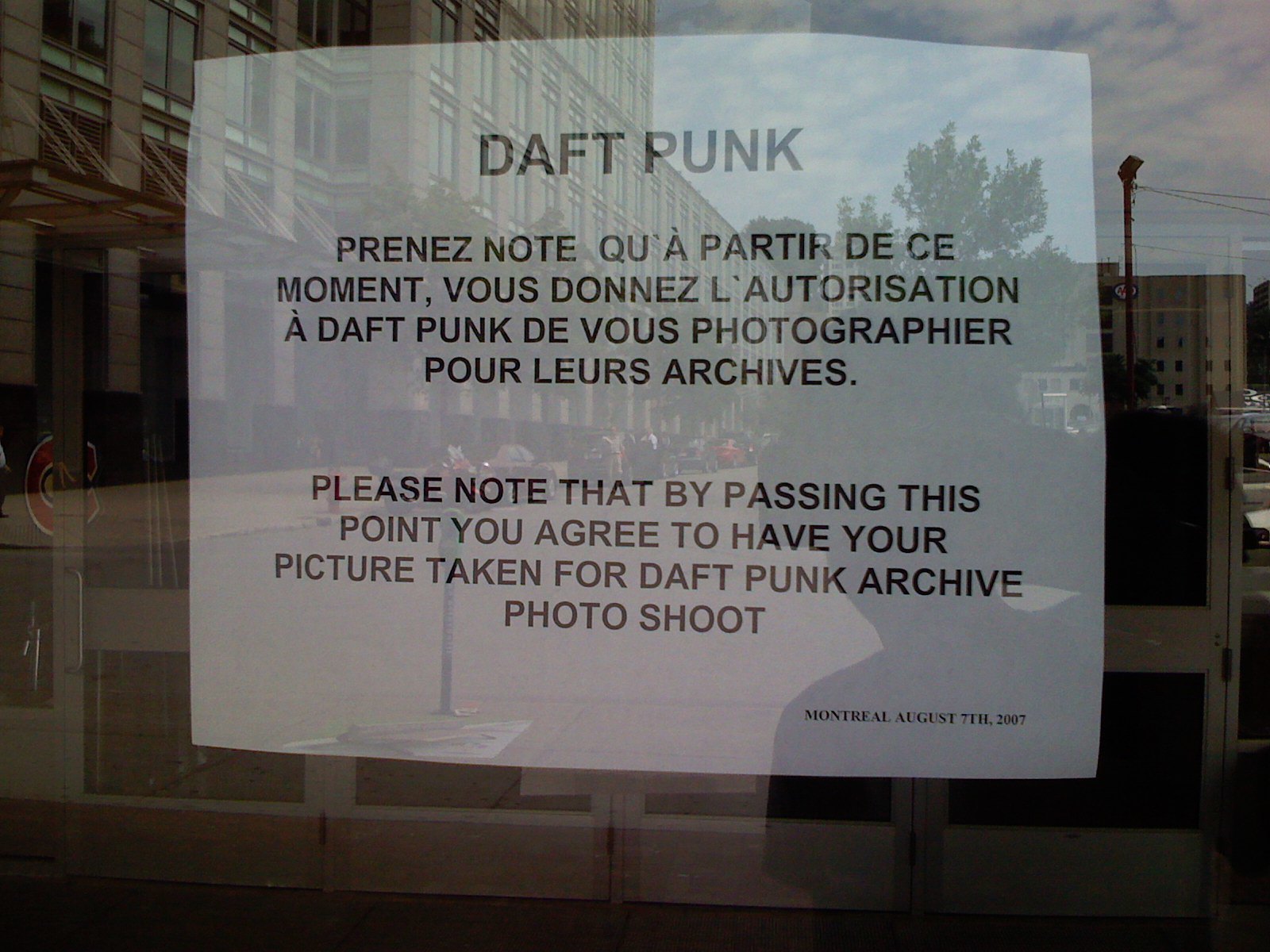In the center of this image, prominently displayed, is a reflective window that captures various outdoor elements such as buildings, power lines, and people. Hanging on the inside of the window is a significant sign, taking up most of the visual focus. The sign, printed on white paper, features the bold text "Daft Punk" at the top, followed by a note in black print: "Please note that by passing this point, you agree to have your picture taken for a Daft Punk archive photoshoot." The bottom-right corner of the sign bears the location and date, "Montreal, August 7th, 2007." The colors visible in the scene include white, black, tan, red, yellow, blue, green, and light blue, contributing to a vibrant and detailed background. The setting suggests the exterior of a store, viewed through the reflective surface of the window where the sign is displayed.